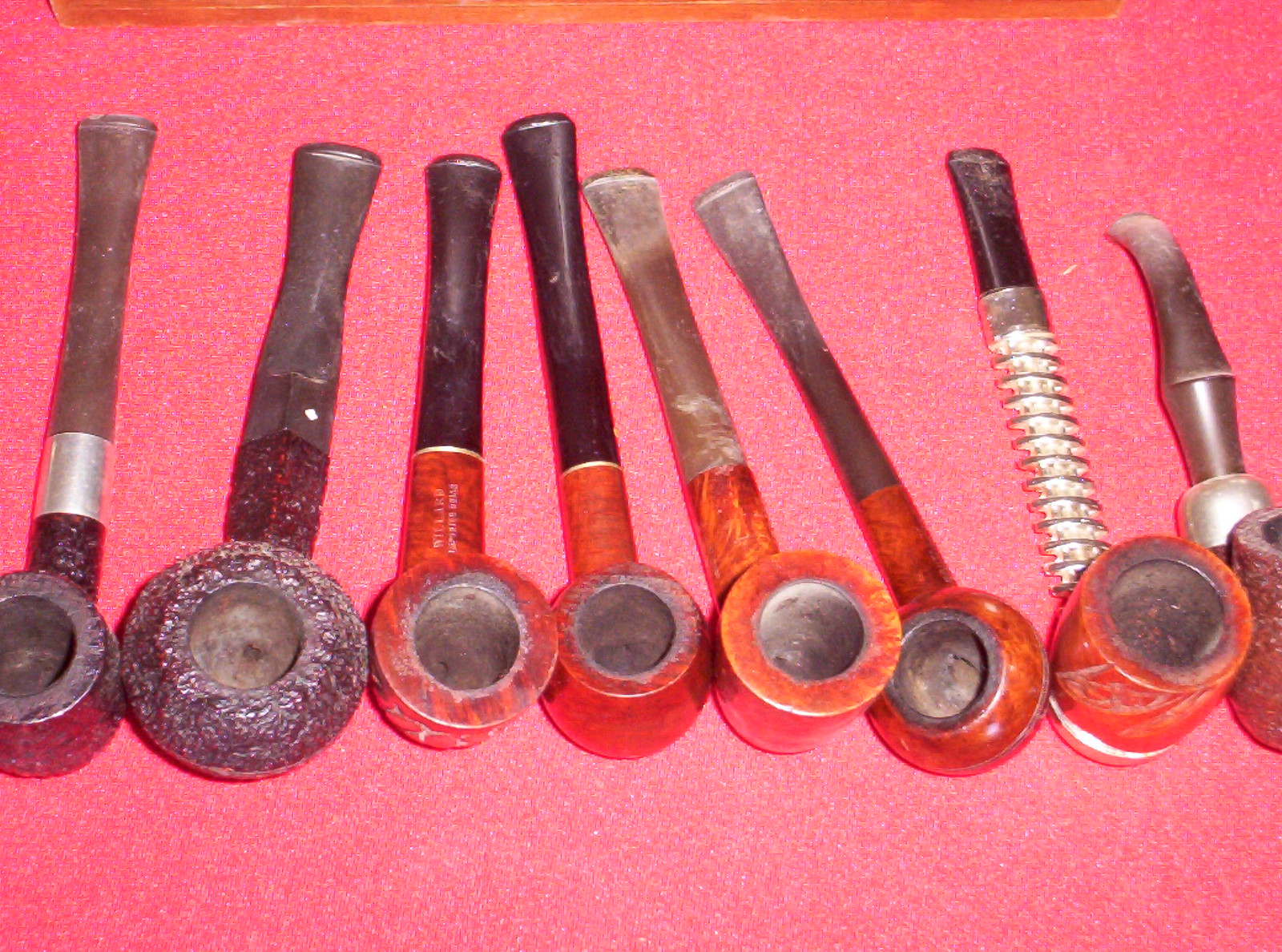The image features a single row of approximately eight tobacco pipes, with their bowls positioned closest to the viewer and their stems and mouthpieces extending toward the top of the frame. The two pipes on the left have darker-colored bowls, while the remaining six exhibit a uniform reddish medium brown hue. Notably, the second pipe from the right stands out with its metallic spiral design along the stem. While the pipes on the left and right edges of the image are partially cut off, their general positioning reveals them to be similar in size with slight variations. The pipes rest on a bright, grainy red surface speckled with small white dots, and a thin strip of brown wood is visible at the top of the image.